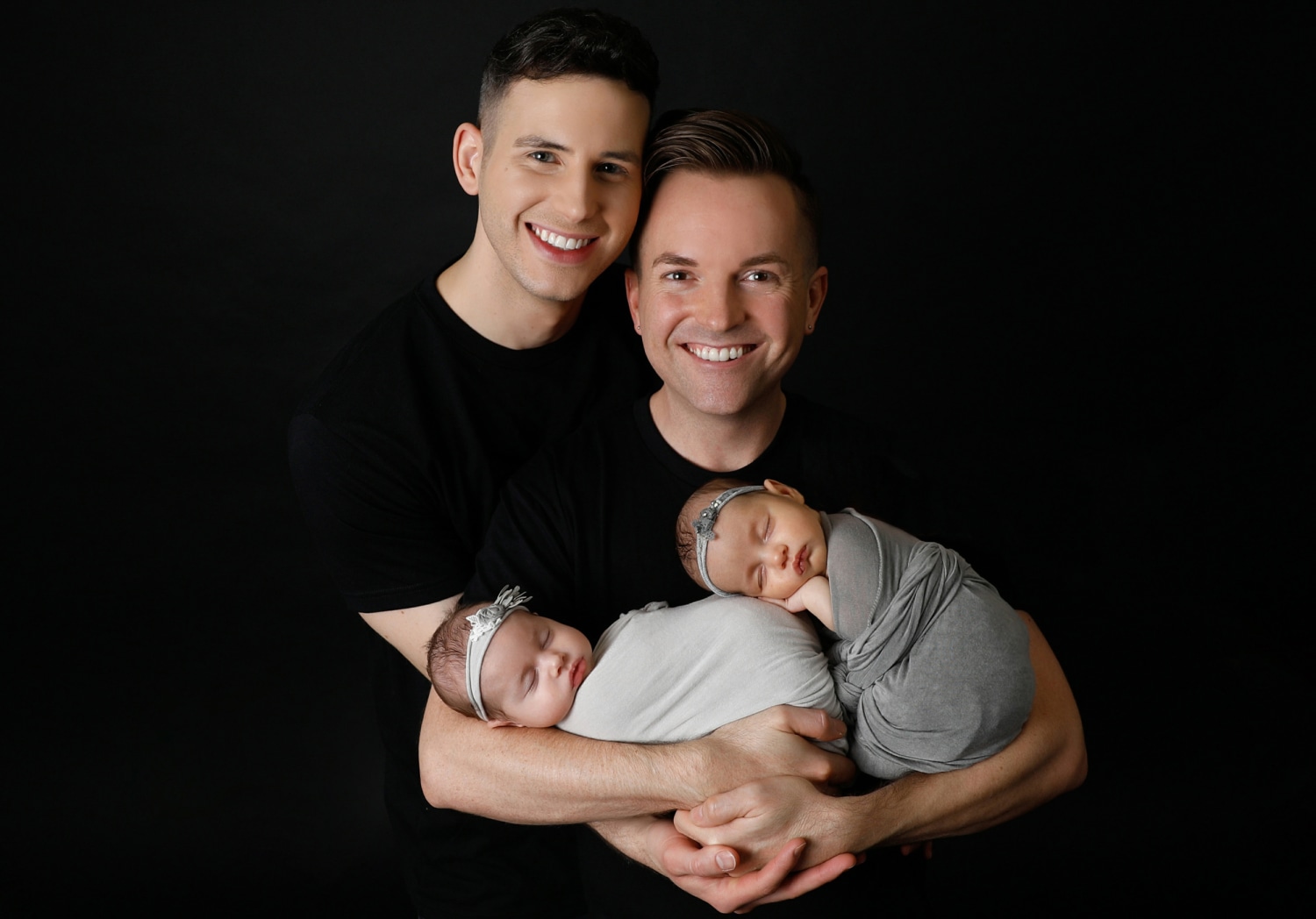In this professionally taken photograph set against a black background, we see a charming family portrait featuring two young men and two adorable infants. The men, dressed in black t-shirts that blend seamlessly with the background, are clean-shaven with nice short haircuts and warm smiles. Their arms are interlocked in front of them, creating a supportive and loving embrace for the two babies they hold. Each baby is swaddled in a light green blanket and adorned with a greenish-blue ribbon around their heads, peacefully asleep in their nurturing arms. The babies' genders are indeterminate in this image due to the neutral colors of their swaddling and ribbons. The black background and attire make the men's smiling faces and the delicate details of the infants stand out, highlighting the tender and intimate moment captured in this almost square photograph. This evocative scene portrays a loving family with two dads proudly cradling their precious little ones.